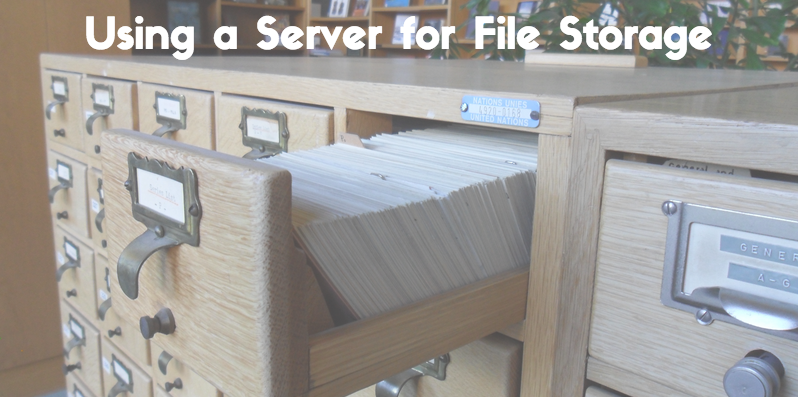This meme-style image humorously titled "Using a Server for File Storage" features a prominently displayed old-fashioned library card catalog system. The caption, written in bold white letters across the top, juxtaposes contemporary digital storage terminology with this retro file storage method. The catalog itself, made of light tan or beechwood, showcases multiple drawers each equipped with small metal brackets and rectangular white label cards. A single drawer in the center is open, revealing neatly arrayed white cards, evoking nostalgia for those familiar with traditional libraries. The background features light brown wooden shelves filled with books, reinforcing the library setting. No people are present in the photograph, allowing full focus on the card catalog and its humorous caption.